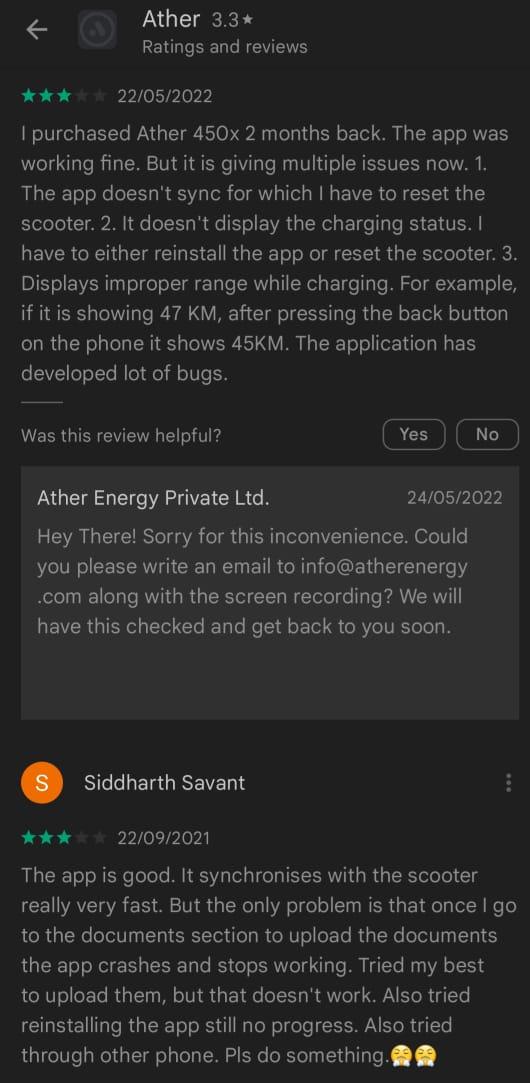The image is a partial screenshot of a phone screen capturing a detailed review of the Ather app, focusing on user ratings and reviews.

- **Top Left Corner**: There is an arrow symbol pointing to the left, followed by a faded gray symbol.
- **Header**: To the right of these symbols, the text "Ather" is prominently displayed, followed by the version number "3.3" and a star icon.
- **Review Section**: The header specifies "Readings and Reviews", with an overall rating of three stars, and the date "22-05-2022".
- **Main Review**: 
  - User mentions they purchased the Ather 450X two months prior.
  - Initially, the app worked well but has since experienced multiple issues.
  - Problems cited include: 
    1. The app failing to sync, necessitating a scooter reset.
    2. Failure to display the charging status.
  - The review continues with additional details regarding the issues.

- **Bottom of Review**: A prompt asks "Was this review helpful?" with "Yes" and "No" buttons located on the right.

- **Additional Information Box**: 
  - Contains the text "Ather Energy Private LTD" followed by a date.

- **Second Review**: 
  - User: Siddharth Savant
  - Rating: Three stars
  - Date: "22-09-2021"
  - Followed by another body paragraph with user comments.

This detailed screenshot captures user feedback, issues with app functionality, and provides the context for the user's experience with the Ather 450X.